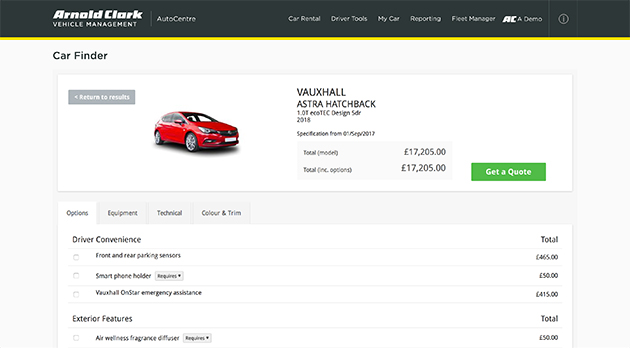At the top left corner of the image, there is the text "Arnold Clark Vehicle Management" in white, and next to it, "Auto Center." Starting from the center and extending to the right side of the image, there are several options listed: "Car Rental," "Driver Tools," "My Car," "Reporting," "Fleet Manager," "AC Demo," and an information icon represented by a lowercase 'i' inside a circle. These elements are positioned above a black strip that spans the top of the image.

Below this black strip is a thin, yellow line. The remainder of the background is white. Below the yellow line, the text "Car Finder" is displayed, followed by a button that says "Return to Results."

Dominating the image is a red, four-door Vauxhall Astra hatchback with the specifications: "1.0 C EOC TEC Design SDR 2018." The poor resolution makes it difficult to decipher some details. Next to the car, there is a price listed in British Pounds, reading £17,205. A green "Get a Quote" button is also visible, inviting users to inquire further about the vehicle.